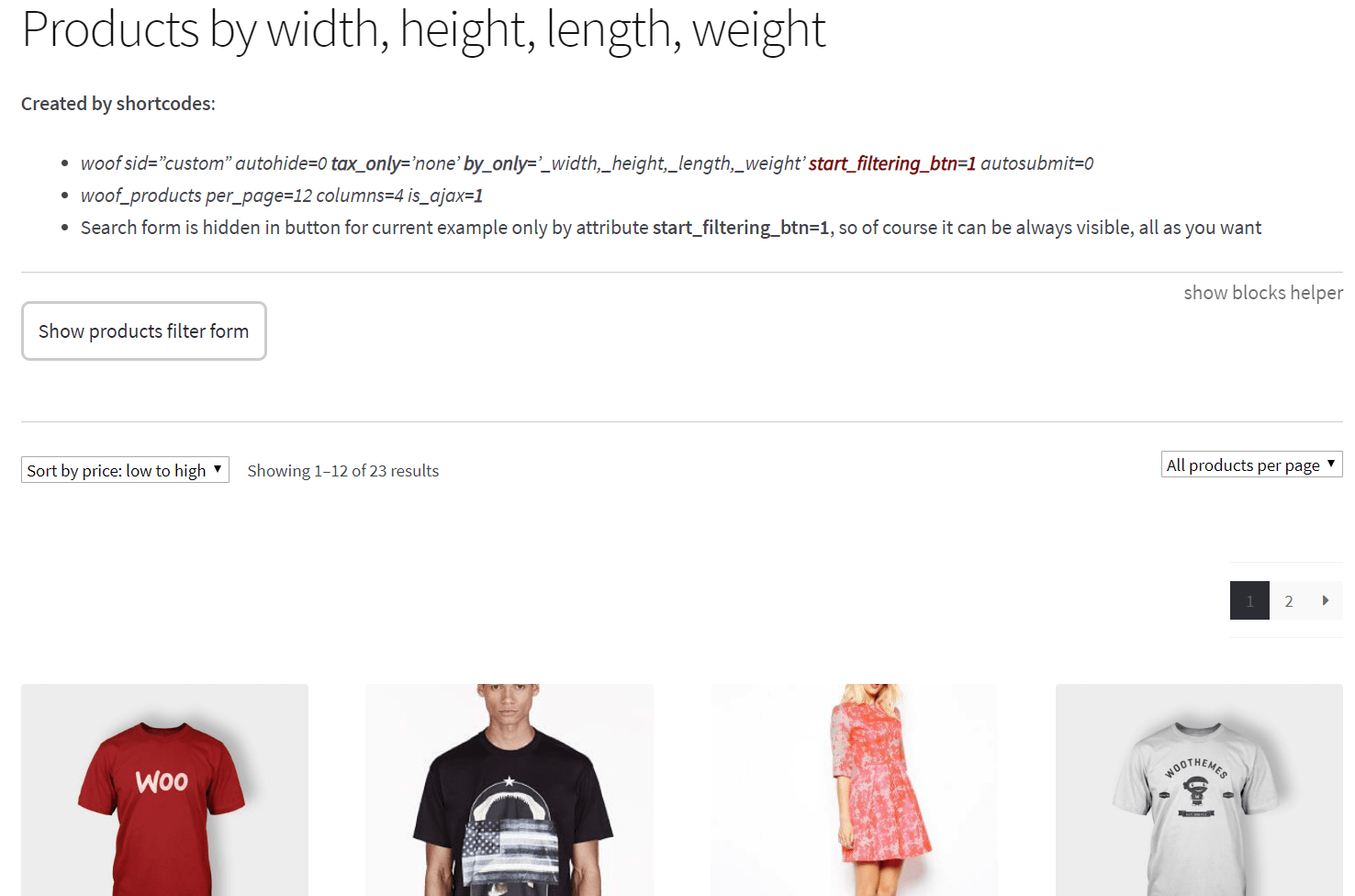This image is a screenshot from an unidentified e-commerce website. The header displays various sorting criteria: "Products by Width, Height, Length, Weight", generated dynamically by shortcodes. Key parameters include custom auto-hide settings, specific taxonomies, unique filtering buttons, and product display configurations—namely twelve items per page arranged in four columns, with AJAX functionality enabled.

The main interface includes a series of filter and sorting options positioned just below the header. Users can engage with buttons labelled "Show Products Filter Form" and "Show Blocks Helper," sort items by price from lowest to highest, and view a pagination feature indicating they are on page one of two, displaying results one to twelve out of a total of twenty-three.

Below these options, four product photographs are showcased. Each product is visually distinctive and positioned side by side:
1. A red short-sleeve t-shirt featuring the word "WOO" in bold white letters on the front.
2. A young man modeling a black t-shirt adorned with a black and gray American flag graphic.
3. A blonde woman in a mid-thigh length pink dress with quarter sleeves.
4. A gray t-shirt emblazoned with "WOO Themes" and a whimsical cartoon ninja illustration.

Overall, the interface provides a streamlined online shopping experience, presenting a variety of clothing items for potential buyers.